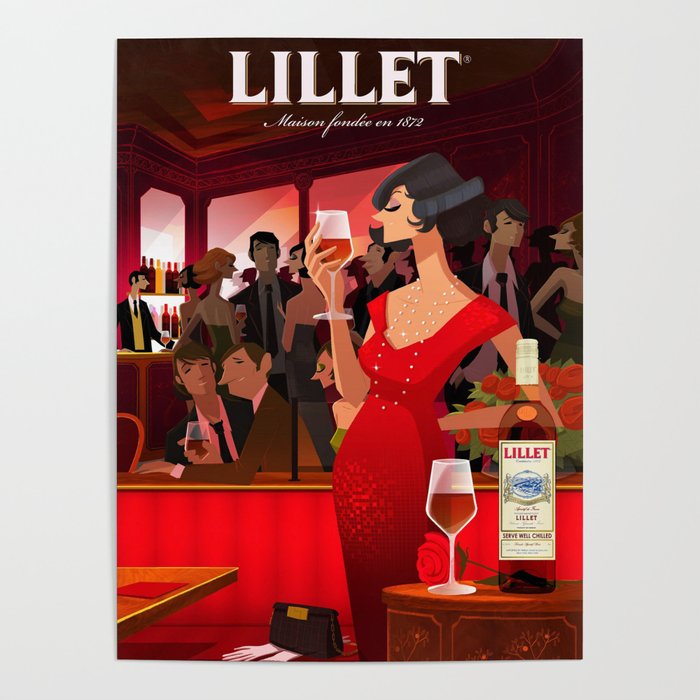This detailed drawing, reminiscent of a 1920s Art Deco advertisement, showcases the alcoholic beverage Lillet, spelled "L-I-L-L-E-T." The advertisement's text at the top reads "Lillet, Maison Fondé, Established 1872" in white block letters and script, indicating the brand's longstanding heritage. The scene is set within a Parisian bar, colored in rich tones of reds, blacks, and grays, bustling with mingling cartoon-like patrons.

At the forefront, a stylish white woman with dark, shoulder-length hair styled in a 1920s bob is the central figure. She dons a striking, low-cut, long red dress and a pearl necklace, holding a wine glass filled with clear brown Lillet in her right hand, poised gracefully in front of her face. Her left hand rests on her hip, adding to her elegant demeanor. In front of her, a brown coffee table displays another glass of Lillet, its bottle, and a red rose, composing an intimate setting.

Supporting the Parisian nightlife ambiance, the background reveals a vibrant bar scene with a bartender attending to numerous bottles and patrons enjoying their evening. A red booth and additional tables, one with a red napkin, add to the setting's authenticity. By her feet, a black purse and a pair of white, elbow-length gloves rest, emphasizing the era's fashion. This meticulously detailed illustration captures the lively and opulent essence of the era in promoting the refined liquor, Lillet.